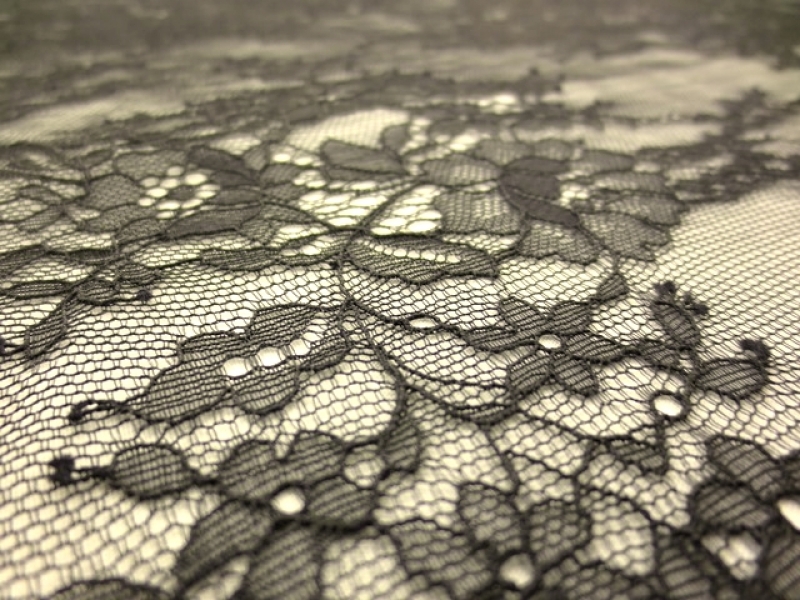This photograph showcases a black lace fabric with a delicate and intricate floral design, stretched out over an off-white or almost flesh-colored surface. The lace features interconnected flowers, leaves, and stems, each meticulously formed by small interlocking circles or hexagon shapes. The floral motifs, sewn with black thread, include round flowers with central holes and teardrop-shaped leaves, some of which are larger and affixed to the stems. The fabric extends from the foreground to the background, where it gradually becomes blurred, emphasizing the detailed pattern in the foreground. The entire black and white image is filled with this ornamental design, giving it a sophisticated and elegant appearance.